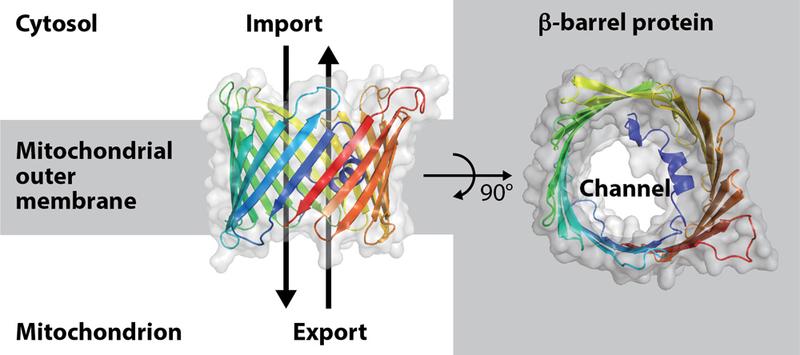The diagram is in a landscape orientation, featuring a white and gray background. In the upper left corner is the term "cytosol" in bold black text. Below this, on a gray bar, is the label "mitochondrial outer membrane," and further down is the word "mitochondrion." Across the white and gray background sections, colored ribbons in blue, red, yellow, and green form a helix-like cylinder, creating a basket-weave pattern with white puffy shapes interspersed. Above and below this structure, the words "import" and "export" are present with two-way arrows indicating direction—one pointing downward, the other upward. To the right, a 90-degree rotation of the cylinder reveals an overhead view labeled "beta-barrel protein" at the top and "channel" in the center, set against a white textured background. The ribbons' colors and orientations remain consistent throughout, suggesting the passage of molecules or ions.